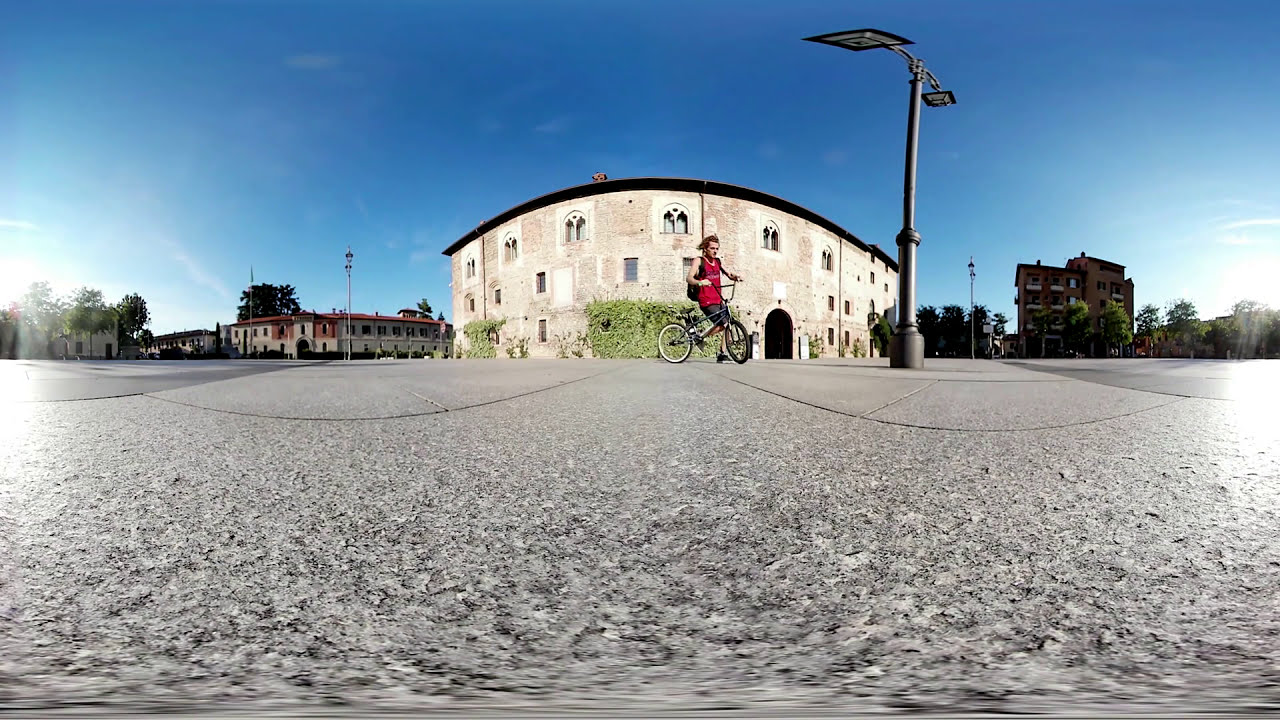In this color photograph, captured with a fisheye lens in landscape orientation, a young man rides his bicycle through a sunny, summer day in a historical European town. The central focus is the young man, wearing a red tank top and shorts, indicating the warmth of the season. He is pedaling along a concrete street with no visible traffic, suggesting it might be early in the day. The image is panoramic, composed of three sections. 

On the left, there is a courtyard bordered by two-story beige and brown buildings, with a few trees behind them. Centered in the photograph, the young cyclist passes in front of a significant three-story light brick building. This architectural landmark boasts numerous arch-shaped and rectangular windows, with a wide, dark archway at the base, possibly an entrance. The scene is punctuated by an overhead floodlight on a pole to the right of this edifice.

To the right, the panorama continues with a taller, four-story red brick building, surrounded by greenery and trees. The photograph portrays a lively, picturesque town bathed in sunlight, highlighting old European architectural features against a backdrop of blue skies. The detailed depiction suggests a blend of representational realism, enriched by the expansive, sweeping view of the town.